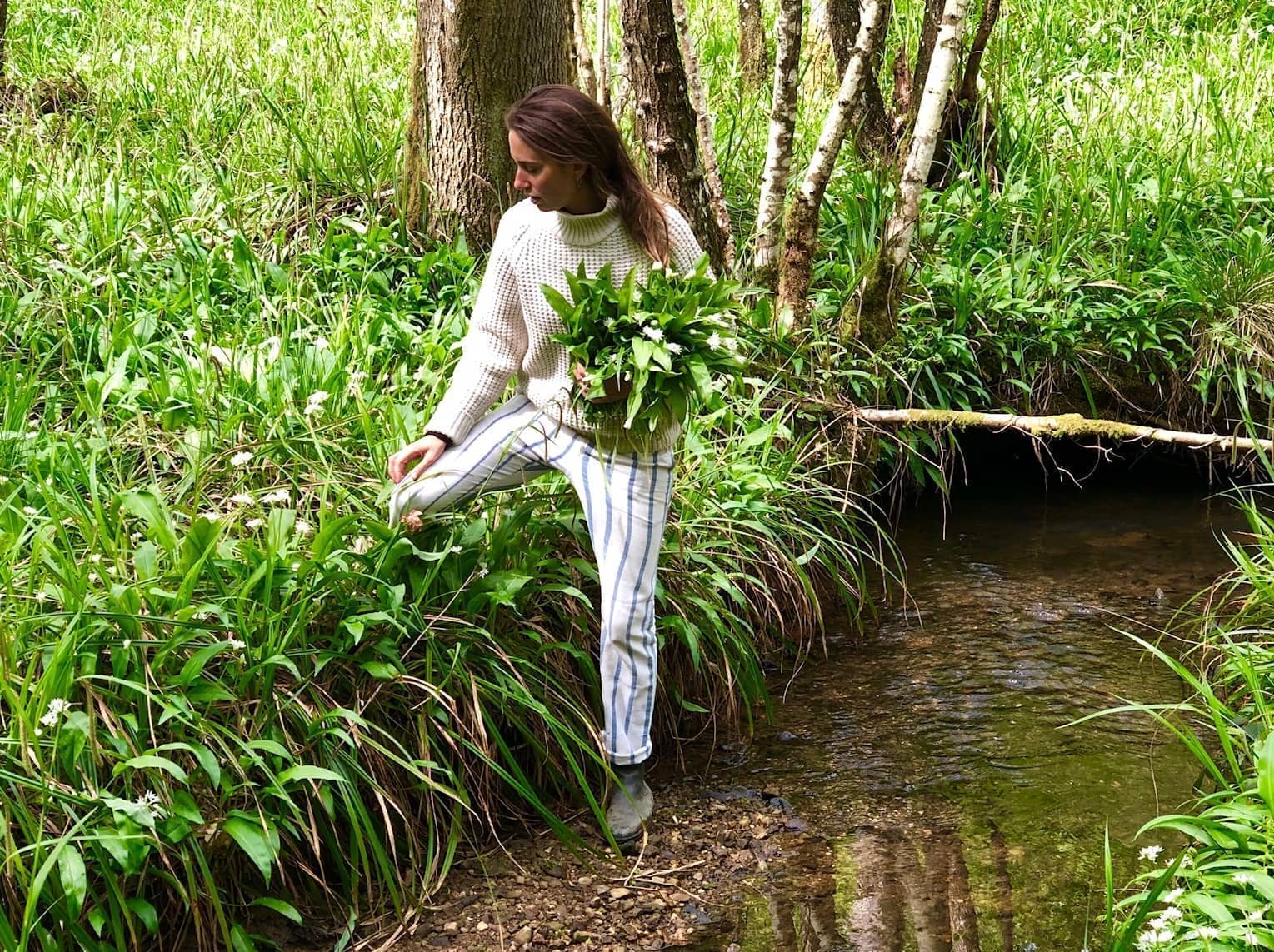In the photo, a woman with long, flowing dark brown hair stands in a lush green forest, one foot immersed in a shallow creek and the other resting on the grassy creek bank. She is wearing a thick white turtleneck sweater and blue-and-white striped pants tucked into boots, suggesting practical yet stylish attire for outdoor activity. The woman is in the midst of gathering plants, cradling a full basket of foliage in her left arm, which includes various grasses, perhaps flax, collected from the edges of the creek. The background is rich with tall, green plants, shrubs, and an assortment of trees, including some that might be birch. A small tree has fallen across the creek, adding a natural element to the serene and verdant scene. Her posture suggests concentration, as she looks down to her right, actively picking more plants from the creek’s bank.